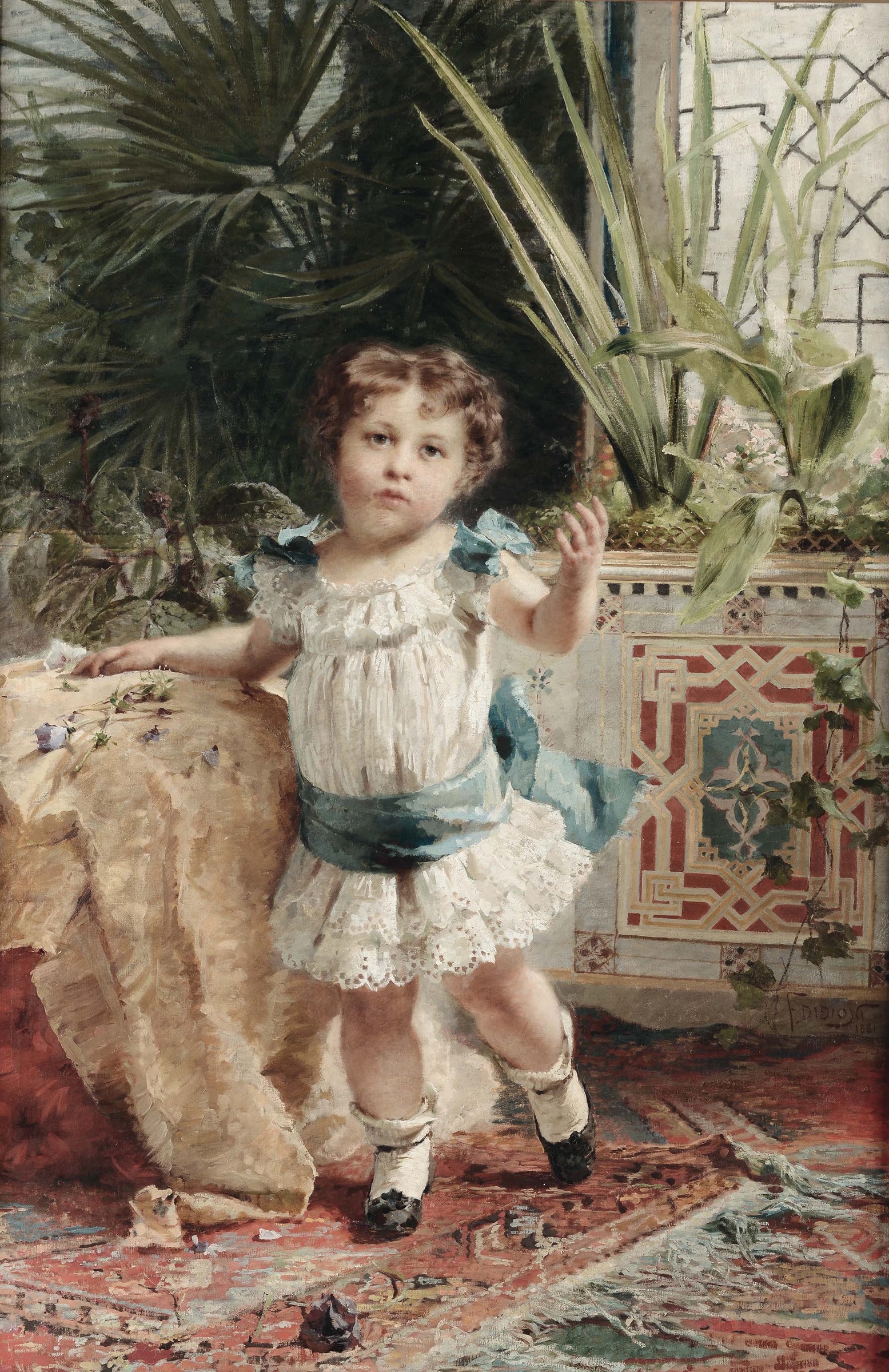This detailed painting, done in watercolors, captures an indoor scene featuring a very young girl, likely a toddler aged around 3 or 4 years old. The child, with very pale skin, stands in the center of the image, her body slightly turned to the left while her head tilts to the right, looking upwards with big brown eyes. She has short, curly hair parted in the middle and rosy cheeks. The girl is adorned in a white, lacy frilled dress, featuring delicate frills at the bottom and on the shoulders. Each shoulder is accented with blue bows, complemented by a blue ribbon tied around her lower waist that is knotted at the back. Her outfit is completed with white socks and little black Mary Jane shoes.

Her left arm is bent with the hand lifted, and her right hand rests on a footstool draped with a white blanket and decorated with a few purple flowers. The floor beneath her is covered with a red Persian rug accented by a white fringe. In the backdrop, lush indoor plants, including large palm plants positioned in the upper left corner and ferns likely situated to the right, add a vivid touch of greenery. Additionally, a tiled square vase brimming with more plants can be seen in the background.

The painting is unsigned except for an elusive artist's signature at the bottom right corner, starting with an "F." Despite its smudged appearance, the artwork bears some resemblance to the style of John Singer Sargent and appears to be at least 200 years old.